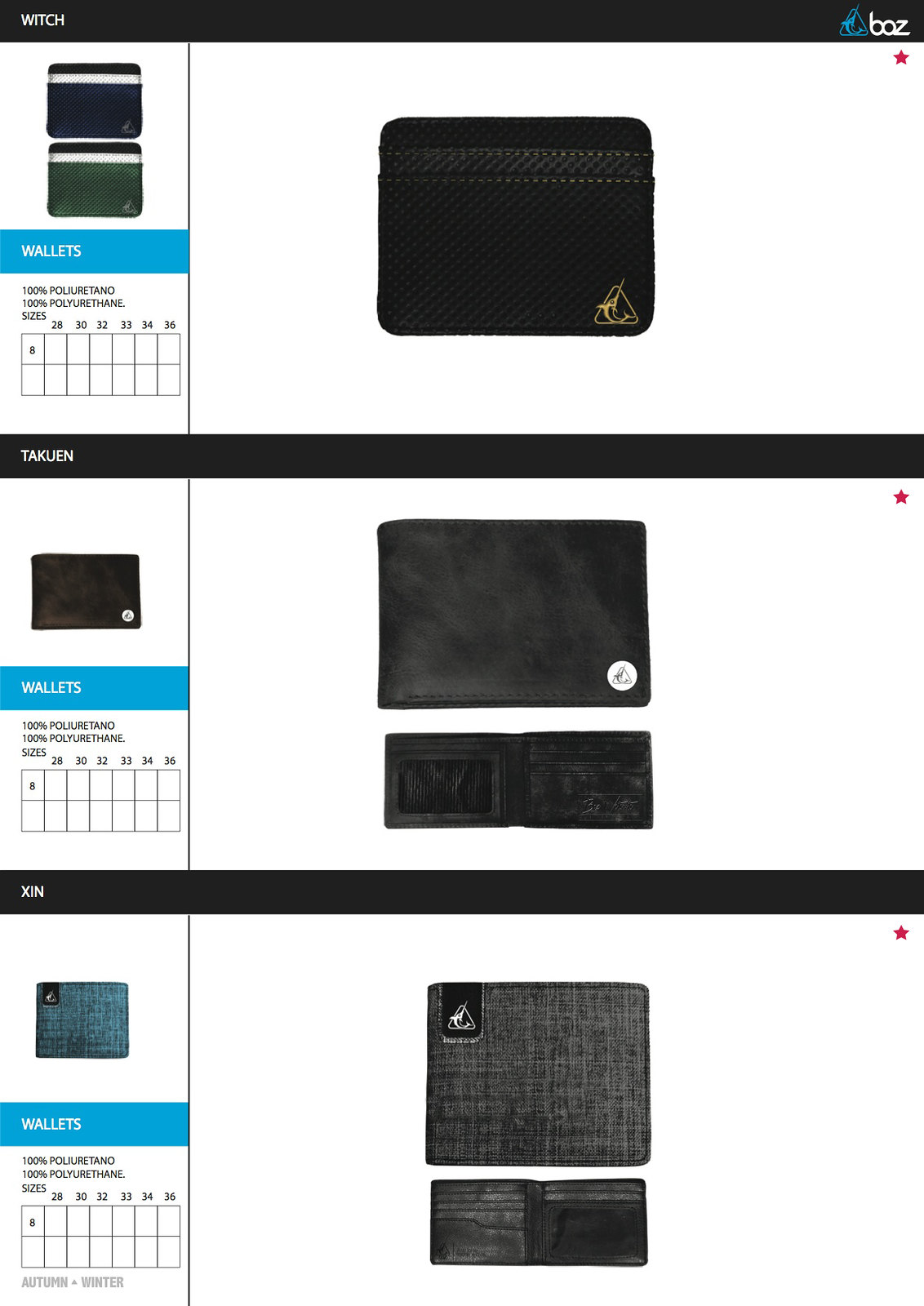This image shows a product page from a website featuring three different wallets arranged in a column. Each wallet belongs to the same brand, identified by a narwhal inside a triangle logo. From top to bottom, they are named "Witch," "Techwind," and "Shin." 

The "Witch" wallet, positioned at the top, is primarily black with a checkered band across the top. It features a cloth-like material and a design element of a swordfish within a yellow triangle on the bottom right corner. Color variations include black, blue, and green.

The middle wallet, "Techwind," is a smooth black leather with a small mountain logo in the bottom right corner, and it is also available in brown. This wallet has a plain, minimalistic appearance.

The "Shin" wallet at the bottom showcases a dark gray denim pattern, though it is also offered in a turquoise blue color. There's a small mountain logo in the top left corner, indicating a possible consistency with the logo design across different wallets. 

Adjacent to the column of wallets is a rating table or measurement chart that provides details about each wallet's capacity and other features, aiding the user's decision-making process, though the text appears slightly blurred.